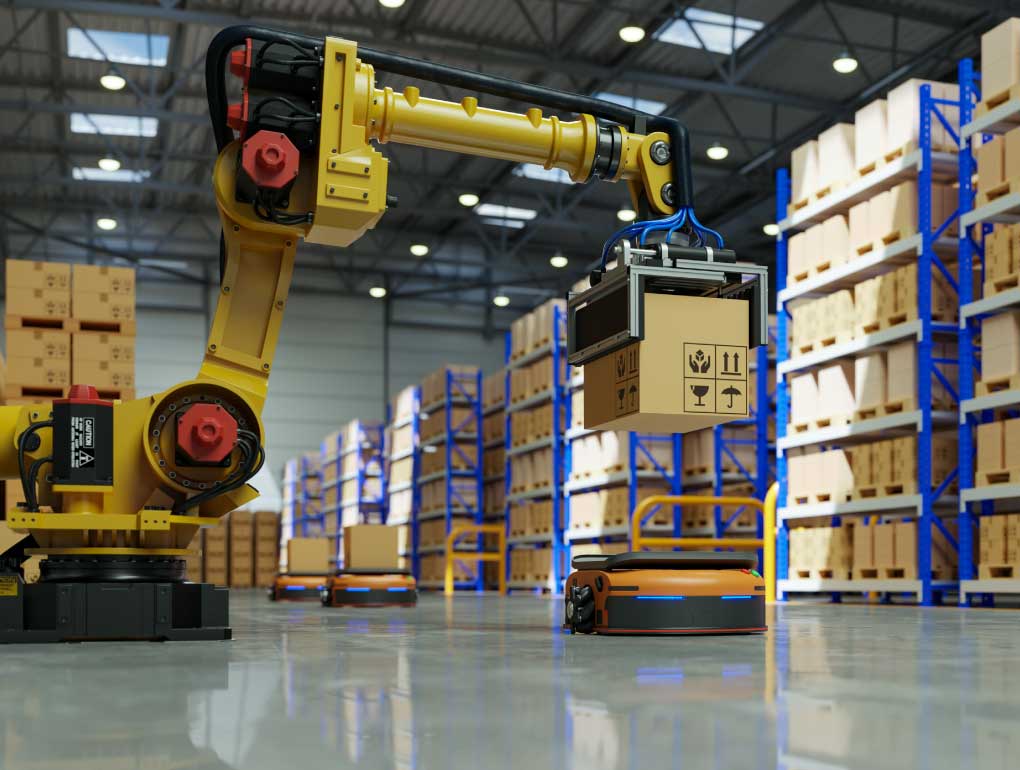Inside the warehouse, a meticulously polished linoleum floor gleams under the industrial lighting. Towering shelves, stacked with neatly lined boxes, stretch high above, creating endless rows of stored inventory. A prominent robot, imposing in size, stands out against this orderly backdrop. Mounted on a robust black platform, the robot's mostly bright yellow body is accented with red knobs and various black components. Resembling a mechanical arm on a motor, the robot is in the process of carefully placing a heavy box onto a scale. In the background, other boxes can be seen similarly positioned on scales, indicating a systematic process of weighing and measuring within the warehouse.